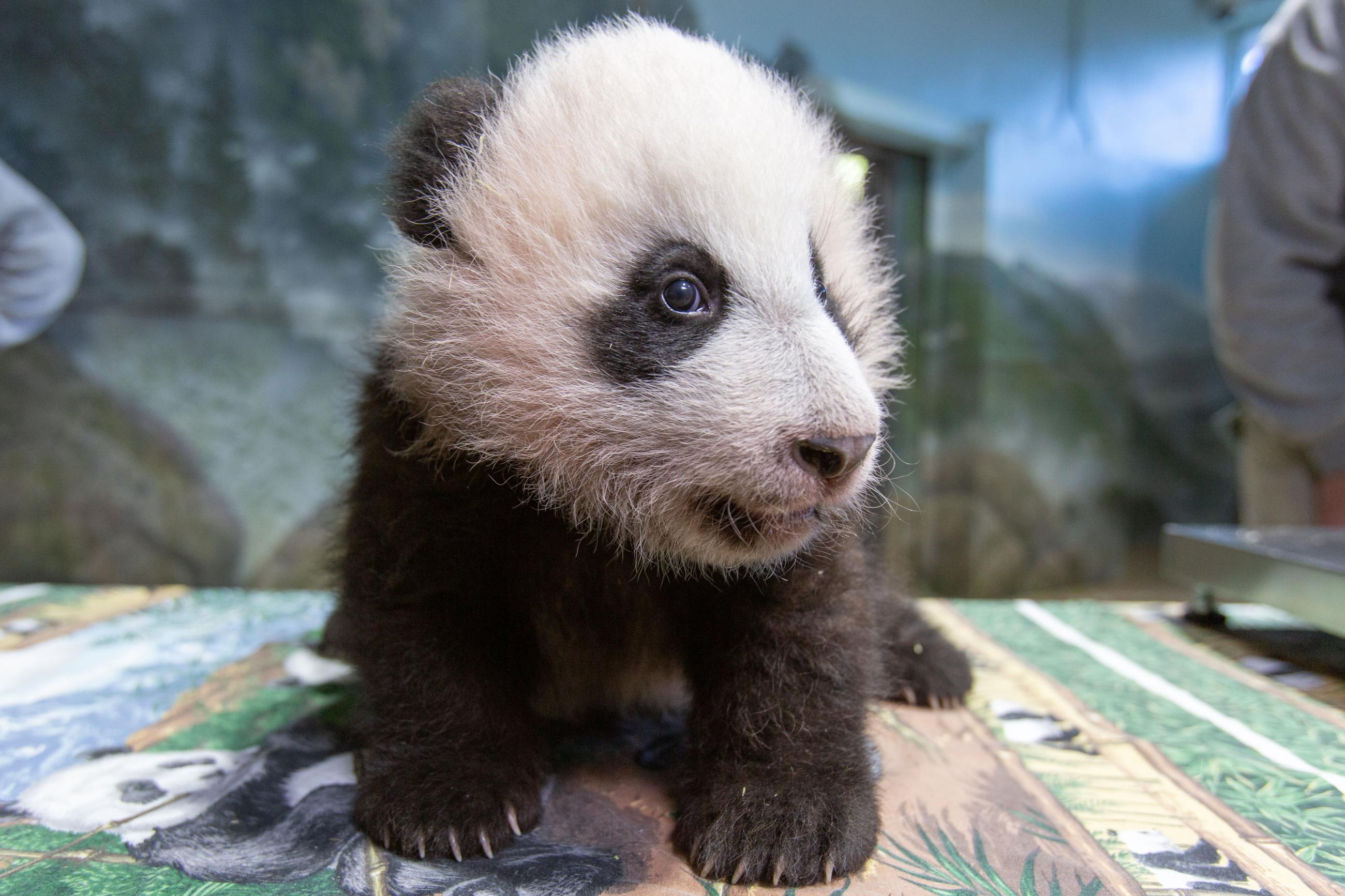In this detailed image, a baby panda with a traditional black-and-white coat is prominently featured. Its fur is lush but not particularly clean. The panda's head is white, with black patches around its eyes, a black nose, and black ears. The baby panda is positioned on what appears to be a table adorned with a mat that has designs of pandas and various patterns in green, blue, and tan. Three of its paws are visible, and you can see its sharp claws.

The panda is facing somewhat to the left, giving a clear side profile, including its tiny black eyes. The background is blurry, with hints of a nature-themed mural on the wall and parts of a door visible. There are also what seem to be the body parts of people, possibly zookeepers, on either side—one arm more distant to the left and a closer one to the right.

Given the setting and the mural, it is likely that this photograph was taken indoors at a zoo. The panda mat and the decor suggest a controlled, thematic environment typically found in such institutions.